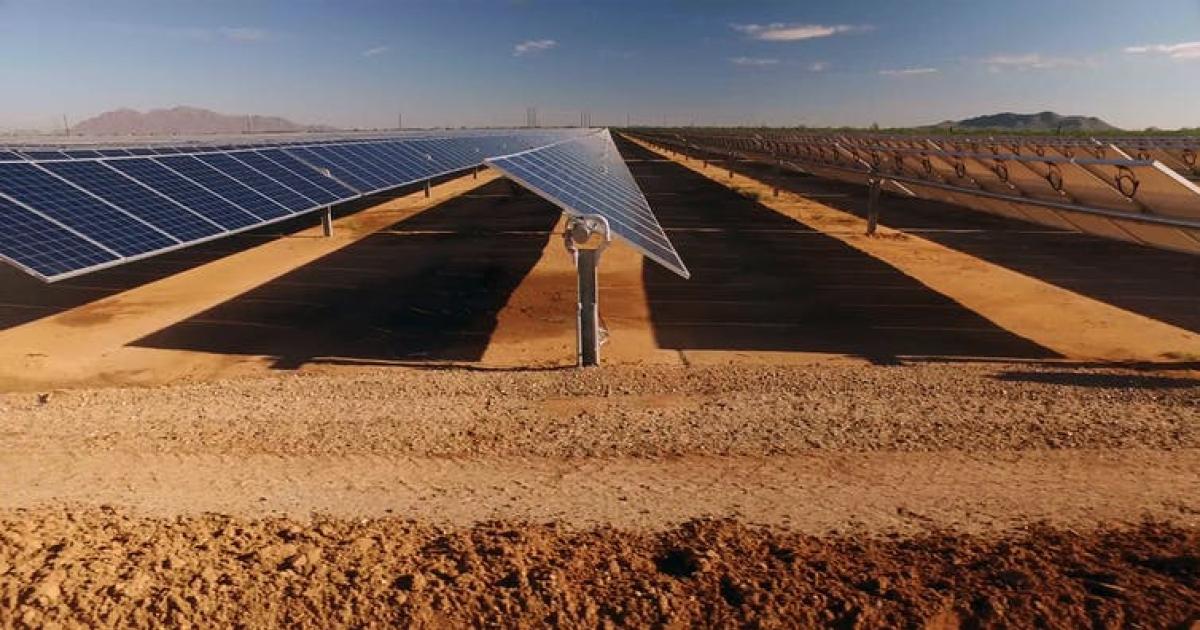In this image, we see an expansive, industrial-scale solar panel array stretching across a vast, dry, desert-like landscape, where the dirt has an orange or reddish clay-like hue. The scene is set under a brilliant blue sky, mostly clear but with a few scattered clouds. Rows of shiny, black solar panels, each framed in white or metal, are neatly arranged in a grid pattern, all angled upwards at approximately 45 degrees towards the top right. The solar panels appear newly installed, and their metal supports cast shadows across the flat, clayey dirt below. Off in the distance, the horizon is adorned by imposing mountain ranges, primarily brown in color, visible at both the far left and far right. Some sparse patches of grass can be seen in the far distance, indicating the sparse vegetation typical of this sun-drenched environment. The entire scene is illuminated by bright daylight, emphasizing the solar panels' purpose of harnessing the sun's energy. The vastness of the array suggests it continues endlessly both vertically and horizontally, underlining the scale of this renewable energy project.